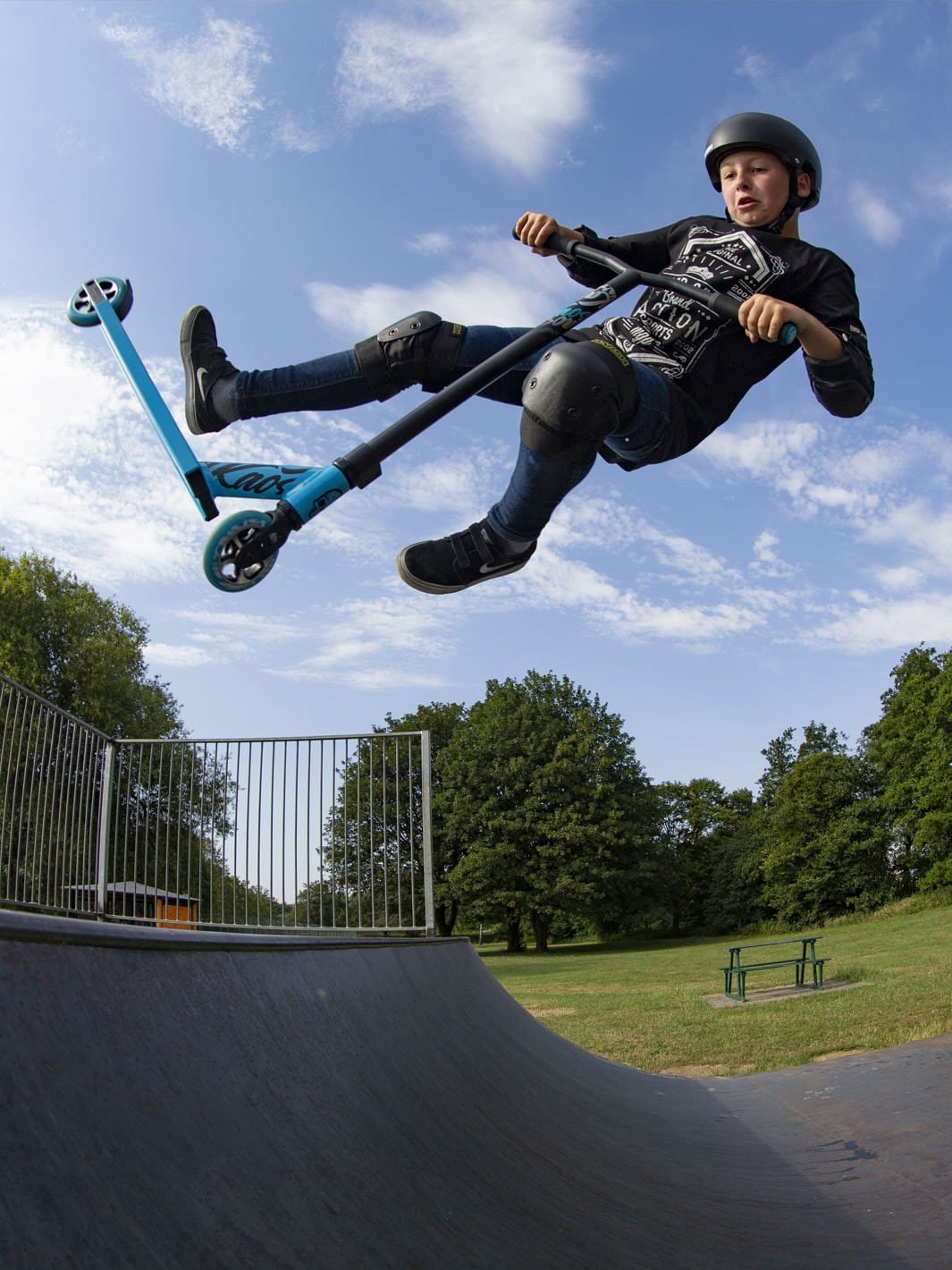This image captures a white boy at a skateboard park, mid-action on a blue scooter as he performs a jump over a black curved skateboard ramp with a metal railing at the top. Wearing a black helmet, black knee and elbow pads, and a black t-shirt with dark blue jeans and black Nike sneakers, the boy is almost horizontally airborne while holding the handlebars of his scooter, his concentrated gaze fixed downward. The park, featuring a picnic table, a green park bench, and green grass with several trees, stretches into the distance where a red building, possibly a restroom, stands to the left. The sky above is a clear blue dotted with white puffy clouds, adding to the serenity of the setting.